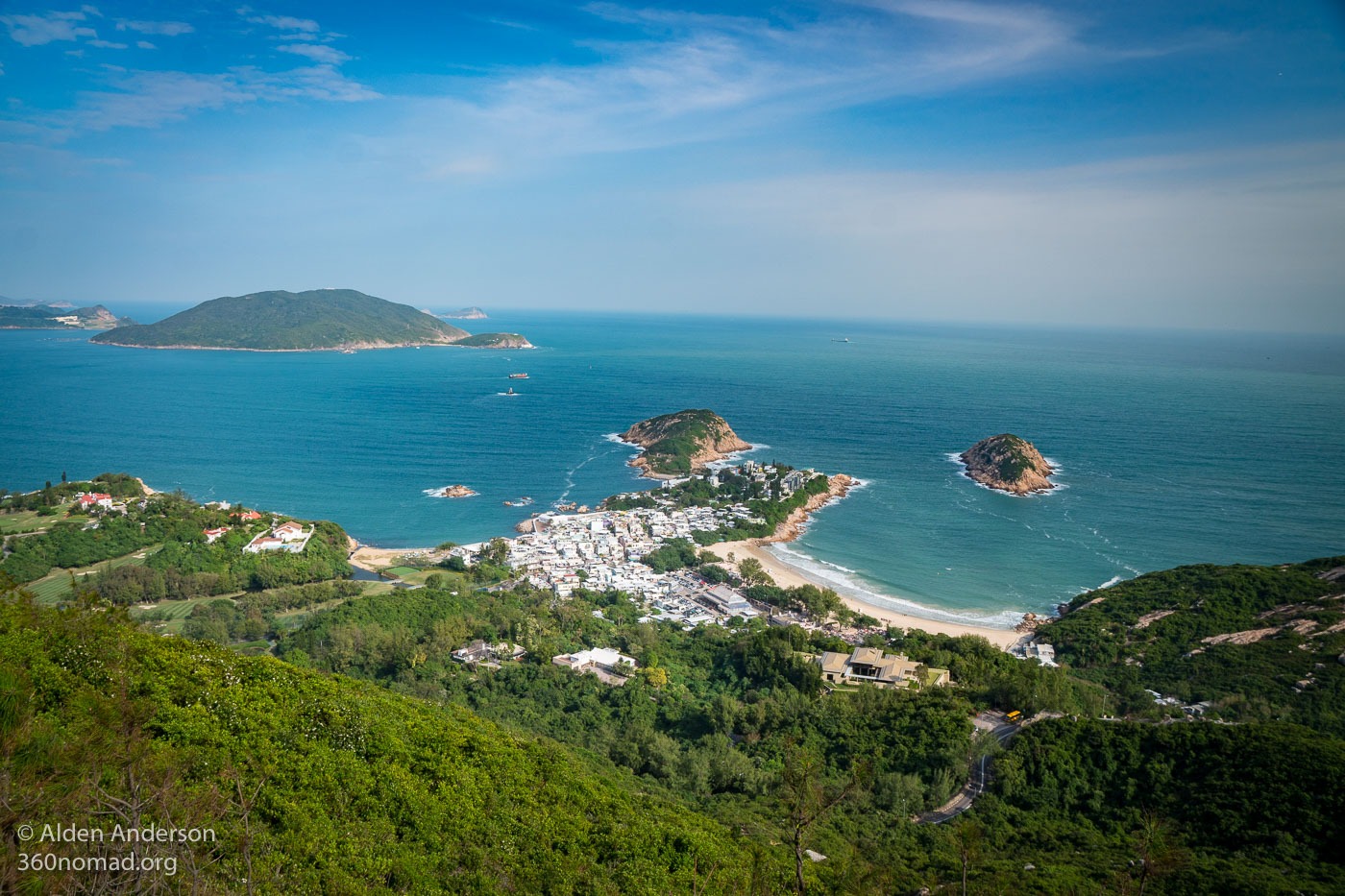This daytime photo captures a scenic and lush outdoor environment, viewed from a hilltop perspective. In the foreground, vibrant green trees and bushes slope downward toward the beach, which features narrow white sand meeting the clear blue and aqua waters of the sea. On the left, a small, distant island covered in greenery rises out of the water, resembling a hill or mountain peak. The middle ground showcases a small community nestled between the beach on the right and another small rocky formation in the calm water. Further to the right, waves gently lap against the shoreline, and a long road stretches along the coast near the town. The bright blue sky is adorned with scattered gray clouds, providing a picturesque backdrop. This image, marked with “oldenanderson360nomad.org” at the bottom, beautifully encapsulates the serene coexistence of land, sea, and sky.